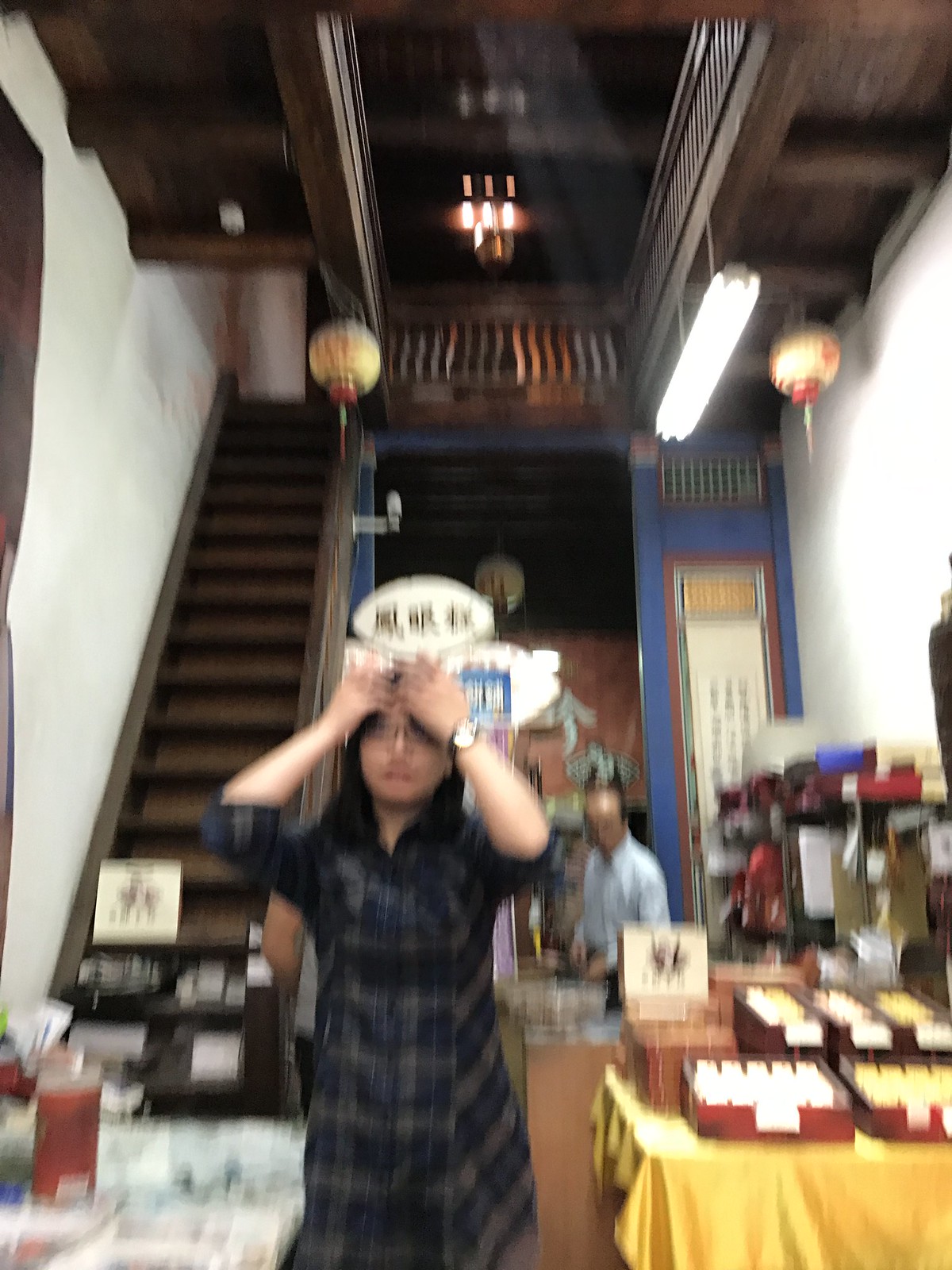The blurry photo captures the interior of a two-story retail store, likely situated in an Asian country, as indicated by the presence of Asian characters and traditional Chinese lanterns. The space has a wooden aesthetic with a tall ceiling featuring two hanging lights—one high above and a lower fluorescent one. A prominent, brown staircase to the left leads to an upper landing area with banisters. In the center of the image, a woman, possibly Asian, stands in a dark plaid dress with checkered patterns. She is adjusting her hair, revealing glasses and a watch with a black band on her left wrist. To her right, a table displaying what appear to be business cards can be seen. In the background, a man in a blue long-sleeve button-up shirt is seated on the ground, seemingly working or organizing items, adding to the bustling, albeit blurry, atmosphere of the store filled with various stationary products.